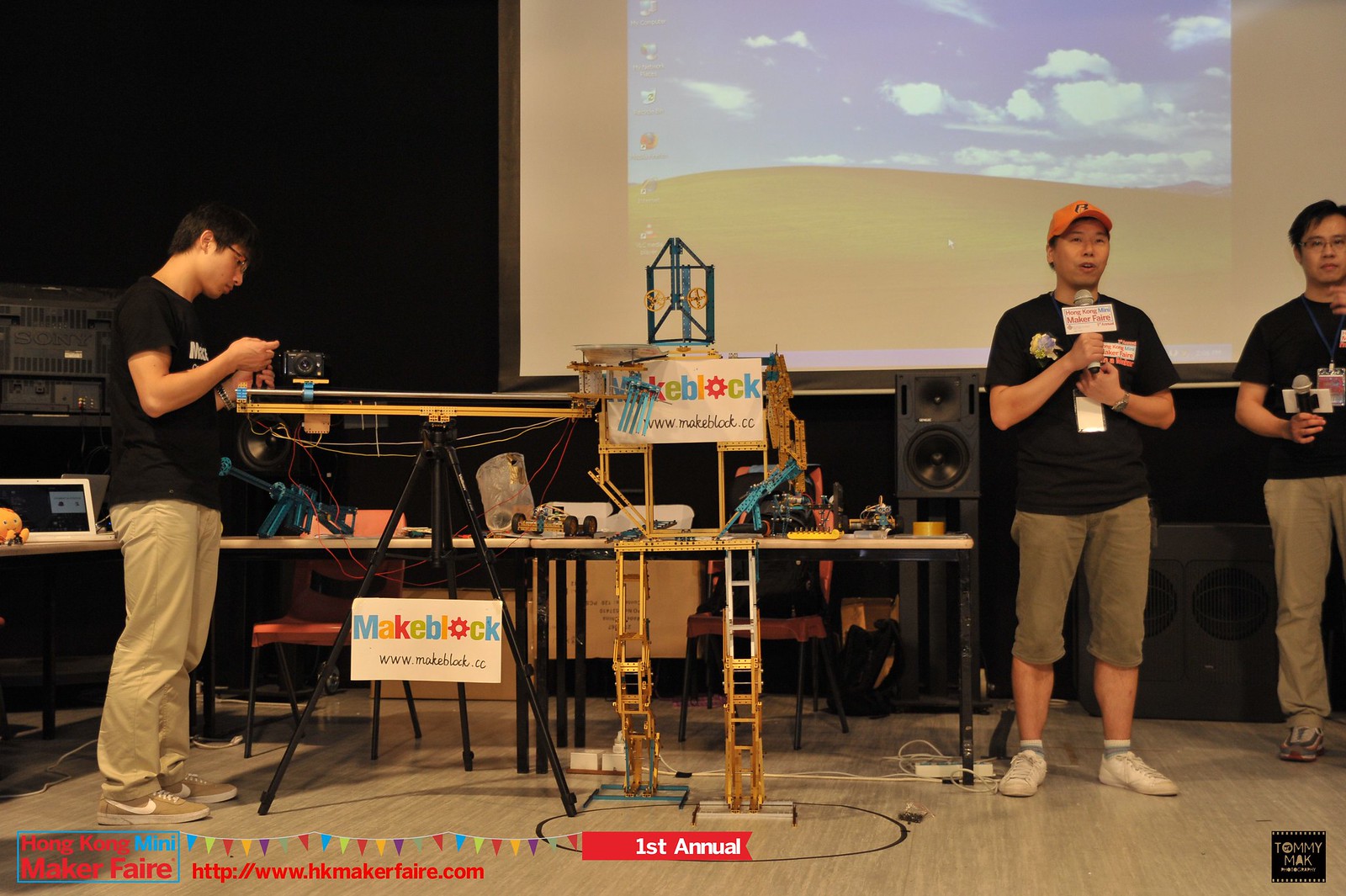The image depicts a presentation at the First Annual Hong Kong Mini Maker Faire, evident from the red ribbon and signs displaying "Makeblock" and "www.makeblock.cc." Three Asian men are showcased prominently, all dressed in black shirts with beige pants and one sporting knee-length shorts and an orange cap. They are equipped with microphones and appear to be showcasing a robotics project that spans both a table and the floor. This project, which is built using wooden components, features blue elements and yellow cogs. Surrounding them is tech equipment, such as speakers and additional gadgets on the table. Behind them, a large projector screen displays a Windows XP desktop, likely providing additional context or details for the audience. The backdrop, wood laminate flooring, and overall indoor setting underscore the bustling, tech-driven atmosphere of this maker fair event.